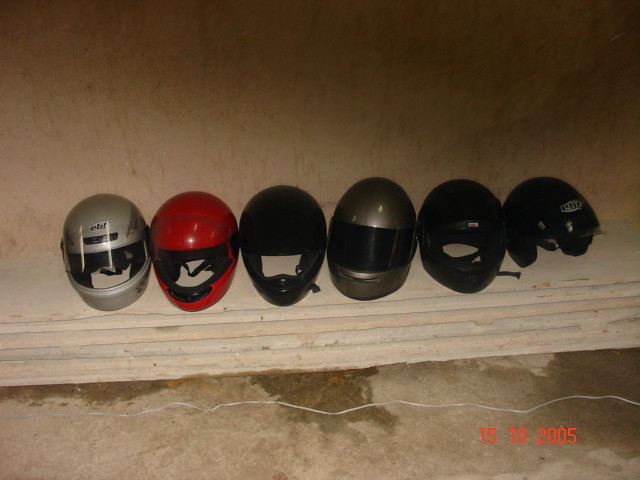This photograph, taken at night, showcases six motorcycle helmets positioned side-by-side on a ledge against a tan-colored wall that appears to have been rained on, causing darker discoloration from raindrops. The setting is outdoors, with the helmets resting on a light-colored ledge above a cement floor that has a noticeable white crack running through it. From left to right, the helmets are: a silver one with a clear shield, a red one with its clear shield up, a black one with its shield up, a charcoal gray one with a thick, black shield, and two additional black helmets with their shields up, featuring black visors. The helmet on the far right is an open-air type, lacking a face shield. A red date stamp reading "15-10-2005" is visible in the bottom right corner of the photograph.